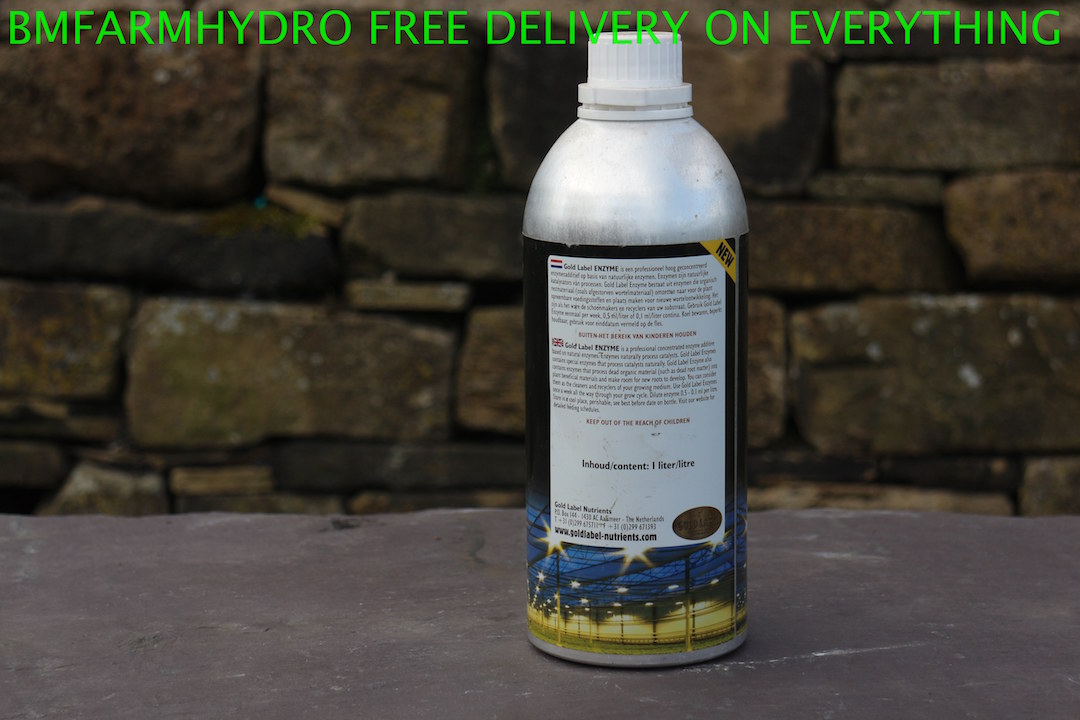This promotional photo features a silver container with a white twist-off cap prominently displayed on a rustic stone platform. The container is labeled with a white and blue design, incorporating a yellow light or element, and is marked with a "NEW" tag on a yellow background on the right side. The label also depicts a cityscape or farm-like visual with blue and yellow elements. Positioned against a backdrop of blurry lay stones, the image emphasizes a natural, earthy theme. Across the top in bold, green capital letters, the text reads "BM Farm Hydro Free Delivery on Everything," highlighting the promotional message.